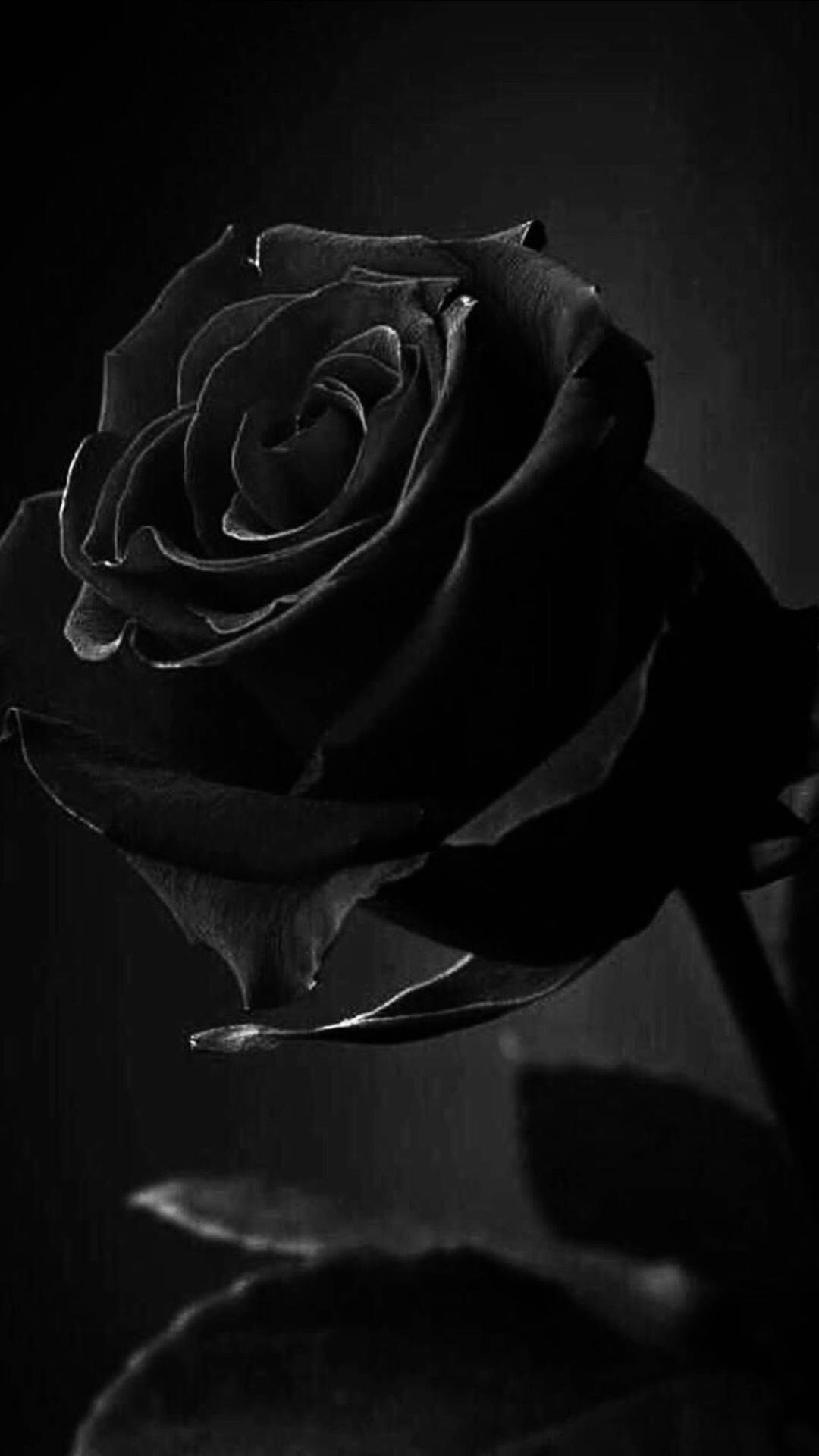This image features a striking black rose at its center, presented in what seems to be a digitally altered or meticulously drawn black-and-white style. The rose stands out sharply amidst the near-absence of light, with its numerous petals arranged in concentric circles. Minimal lighting creates a subtle shine around the petals, especially accentuating the bottom of the flower. The background, an enveloping darkness, makes it difficult to discern additional elements beyond the rose itself. The stem and leaves, though also black, can be distinguished by their shapes and bristly edges. Shadows of the rose and its leaves cast onto an unseen wall provide depth, albeit somewhat blurry. The composition highlights the floral subject, with the rose angled slightly towards the left, making it the unmistakable focal point of this dark, evocative artwork.